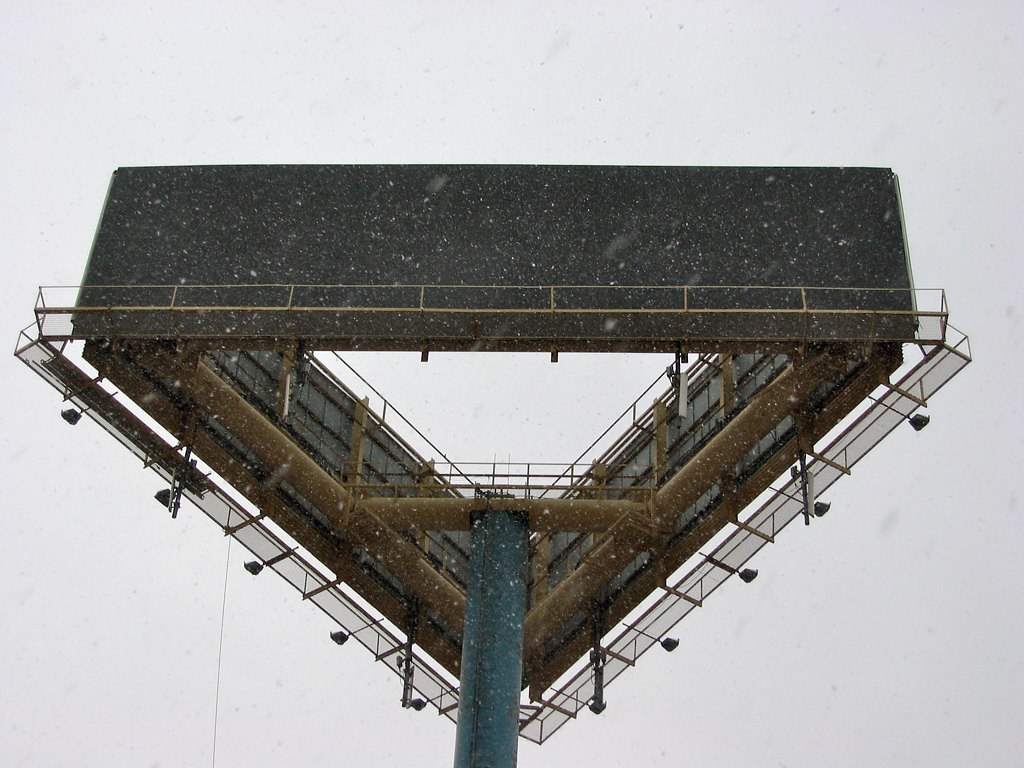The image features a triangular billboard structure viewed from ground level, looking upward. The billboard's triangular shape tapers to a point at the bottom of the image, with the broad base facing the top. The front face of the triangle is a plain black billboard adorn with white spots. Below this, a grayish-brown railing runs horizontally, partially obscuring the lower edge of the base. 

On the sides of the triangle, the backs of the other billboard faces are visible, showcasing a complex metal framework. There is a ledge along the outer edges of these sides that appears see-through, adding to the structural intricacy. Supporting the entire billboard is a thick, blue metal pole that extends upward into the center of the triangle. At the top of the pole, a U-shaped metal structure securely attaches it to the billboard, ensuring the stability of the triangular formation.